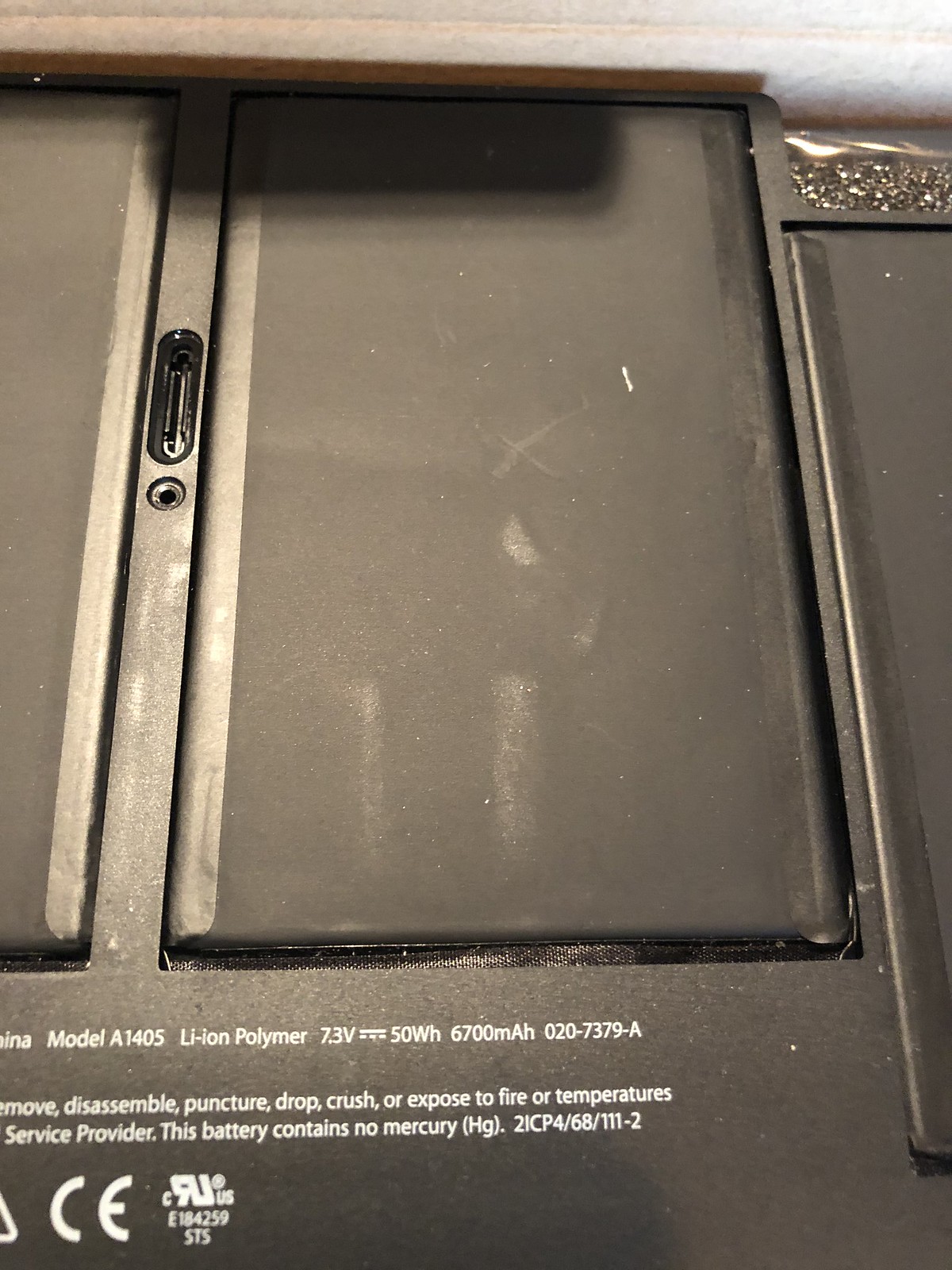This image depicts a close-up, vertically aligned photograph of the inside of an electronic device, likely a laptop or a MacBook, focusing on its battery compartment. The main object, centered and taking up most of the frame, is a rectangular battery, distinguished by its matte black color with visible dust and white particles. The battery specifications are prominently displayed in white text at the bottom and read: "Model A1405 Li-Ion Polymer, 7.3V, 50Wh, 6700mAh, 020-7379-A." Below these, there are partial visibility warnings and usage instructions stating, "Do not remove, disassemble, puncture, drop, crush, or expose to fire or temperatures. This battery contains no mercury." The upper right side of the image has a slight brownish tone and some glitter-like particles. An oval-shaped feature, possibly a card insertion slot, and a small circular area resembling a button are also visible between what appears to be battery compartments or modules. The image's background is minimal, suggesting an indoor setting, but details are indistinct due to the zoomed-in perspective.